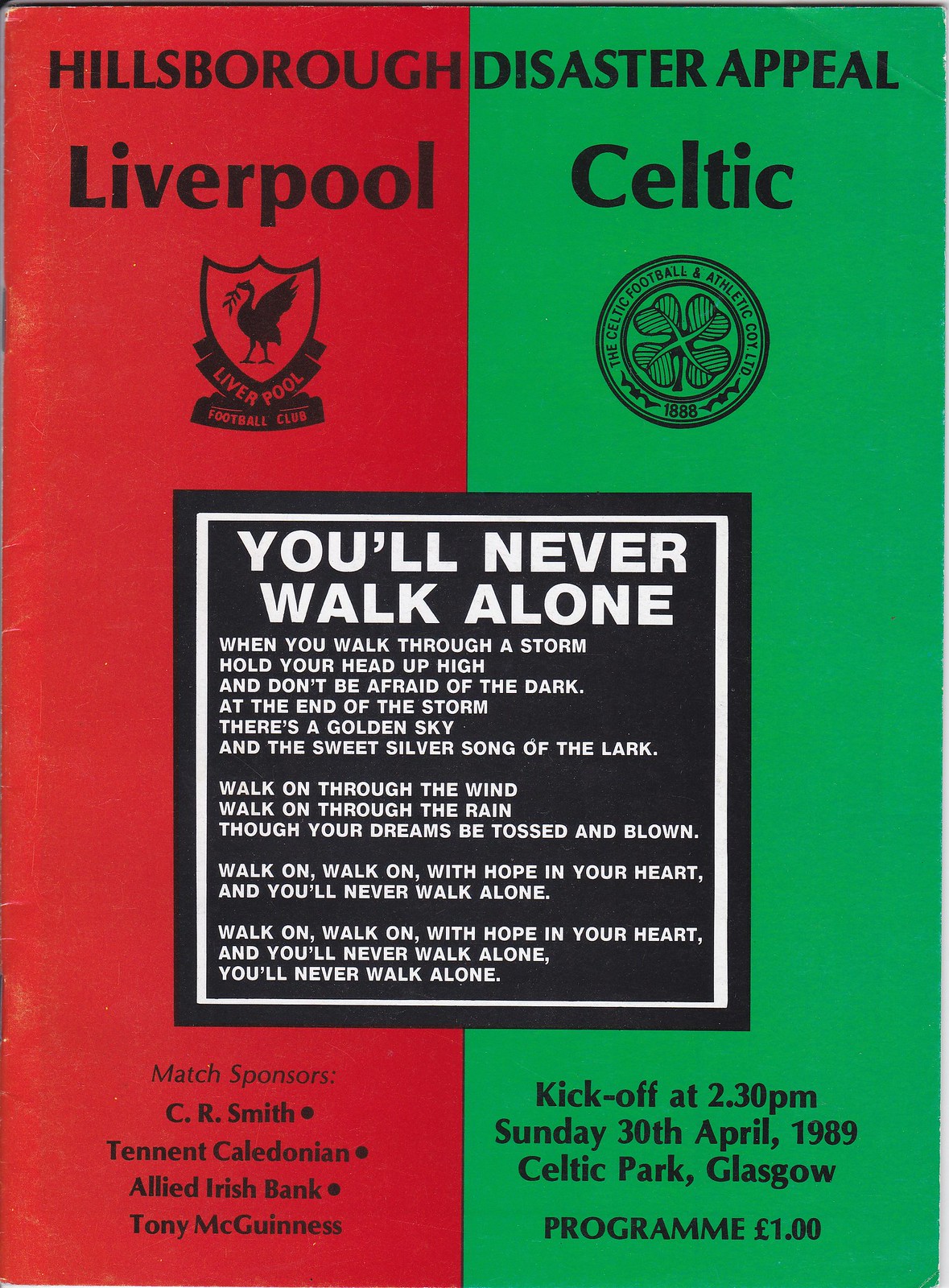The image depicts the front of a football program for a match dedicated to the "Hillsborough Disaster Appeal," dated Sunday, April 30, 1989, at 2:30 p.m., taking place at Celtic Park, Glasgow. It is vertically split into two halves: the left side is red, representing Liverpool, and the right side is Celtic green. The text at the top is in black and declares "Hillsborough Disaster Appeal." Each side features the respective team's name and emblem—Liverpool on the red side with their iconic bird holding a leaf and Celtic on the green side with a shamrock within a circle. Centered on the cover is a large black square with a thin white border, displaying the phrase "You'll Never Walk Alone" in white lettering, followed by the song lyrics:

"When you walk through a storm, hold your head up high, and don't be afraid of the dark. At the end of the storm, there’s a golden sky and the sweet silver song of the lark. Walk on